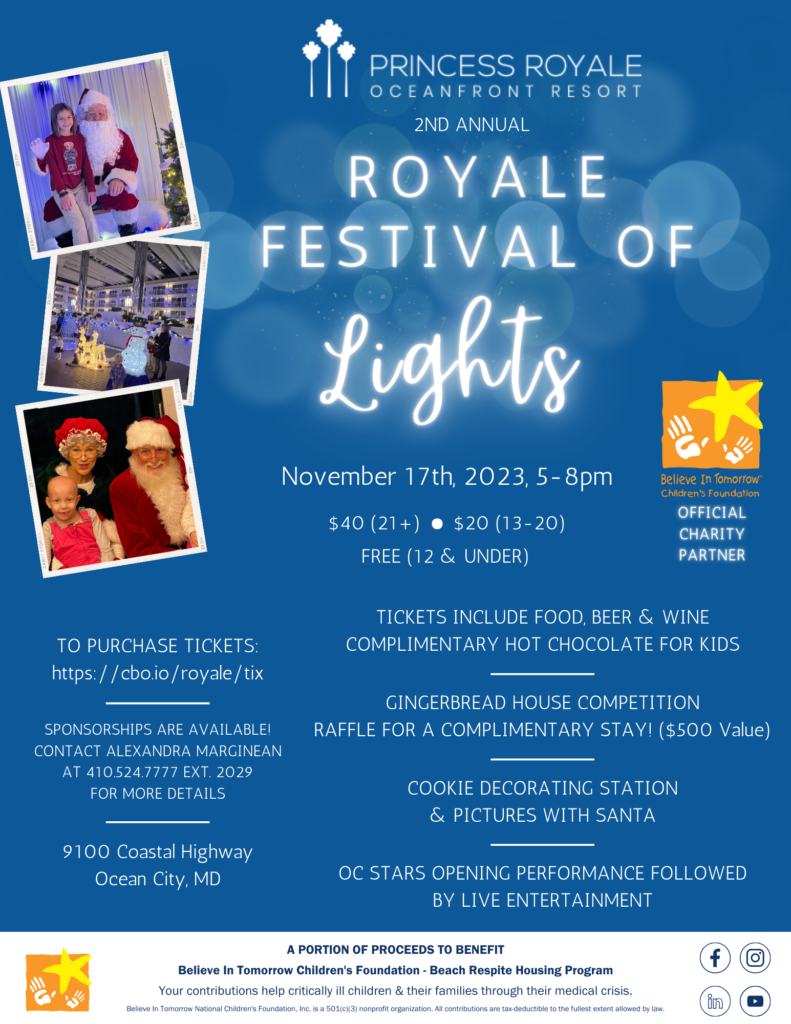This poster for the "Second Annual Royal Festival of Lights" features a blue background adorned with light blue and white dots, reminiscent of blurry holiday lights. On the left side, there are three photos: the top picture shows Santa Claus with a little girl, adorned with Christmas decorations such as a tree and festive lights; the middle photo captures a bald child with Santa and Mrs. Claus, possibly a child with cancer; and the bottom image likely shows a scene with people dancing. At the top right, bold white text announces "Princess Royale Oceanfront Resort" followed by "Second Annual" and “Royal Festival of Lights” in glowing and cursive letters. Below that, it mentions the event date, November 17th, 2023, from 5 to 8 p.m. To the right, there is an orange logo featuring a yellow star with white handprints. The poster also includes detailed information about tickets, food, and competitions, as well as logos, addresses, and social media icons. A white banner at the bottom states, "A portion of proceeds to benefit Believe in Tomorrow Children's Foundation Beach Respite Housing Program," highlighting the event's charitable cause.